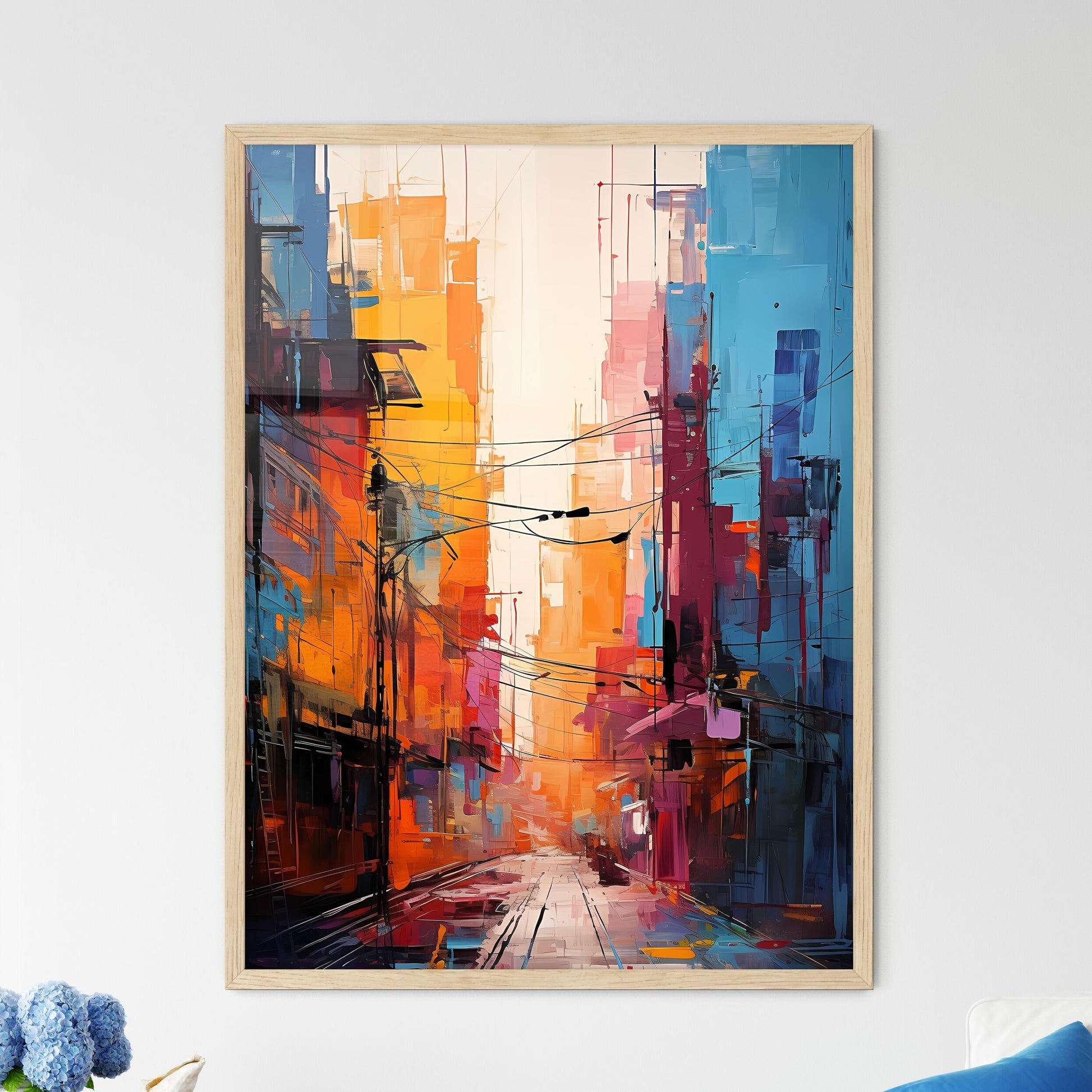This image captures a vibrant and detailed watercolor painting of a city street. The painting offers a front point of view of the street, flanked by an array of colorful skyscrapers in shades of blue, burgundy, orange, yellow, and pink. The medium-tall buildings on the right mainly feature blue and purple hues, while those on the left predominantly showcase oranges and yellows, along with touches of blue. Antennas are visible atop these skyscrapers, and numerous electrical wires stretch across the street from building to building. The street itself, devoid of people or cars, contains lines resembling either lane markers or trolley tracks. Notably, the painting is framed in light gray, and outside the painting, near the bottom left corner, three small circular-based blue flowers and a blue patch can be seen. The scene suggests a daytime setting with a white sky, possibly depicting a shopping or residential district.